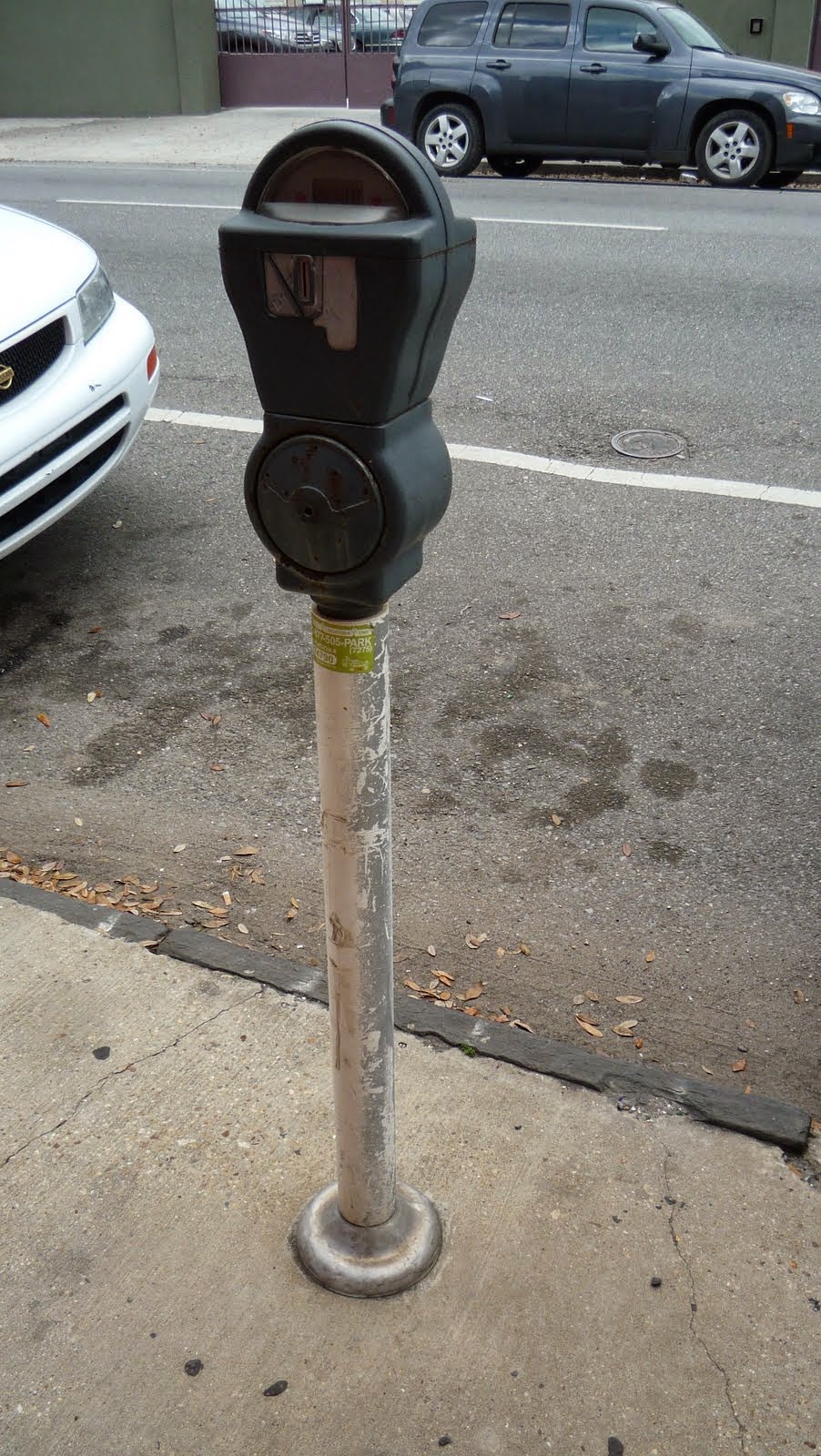This image captures a detailed view of a traditional parking meter prominently positioned on a concrete sidewalk. The parking meter, mounted on a weathered silver metal pole with remnants of white paint, features a dark gray or black body with a rounded top displaying the time left for parking. The placement of coin slots suggests it is designed for quarters. The sidewalk beneath the meter shows signs of age with various oil spots and scattered leaves.

To the left of the meter is the front end of a white car, possibly identifiable as a Nissan. The sidewalk transitions into a black paved road marked by white dashed lines in the center and solid white lines on the edges. Notably, there is an older black or navy blue SUV parked on the opposite side of the street, facing the same direction as the white car, indicating a one-way street. In the background, a notable feature is a green cement wall with a pair of substantial brown metal gates that partially conceal additional parked vehicles. The setting suggests an urban environment with typical street traffic elements and parking provisions.